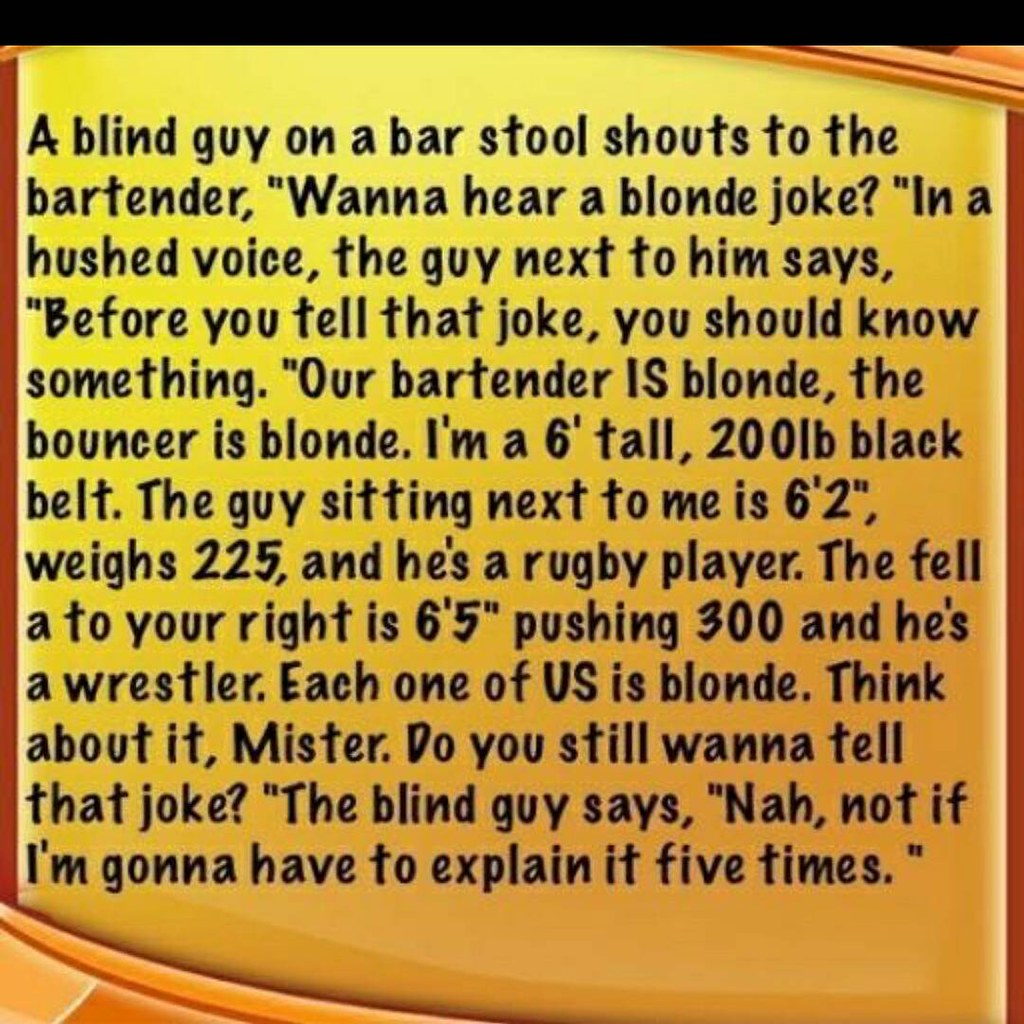The image is a screen grab of a large wall of text set against a yellow gradient background that transitions to orange in the bottom right corner. The text, written in black, reads: "A blind guy on a bar stool shouts to the bartender, 'Wanna hear a blonde joke?' The guy next to him, speaking in a hushed voice, says, 'Before you tell that joke you should know something. Our bartender is blonde, the bouncer is blonde, and I'm a six-foot-tall, 200-pound black belt. The guy sitting next to me is six-foot-two, weighs 225 pounds, and he's a rugby player. The fellow to your right is six-foot-five, pushing 300 pounds, and he's a wrestler. Each one of us is blonde. Think about it, mister. Do you still want to tell that joke?' The blind guy responds, 'Nah, not if I have to explain it five times.'"